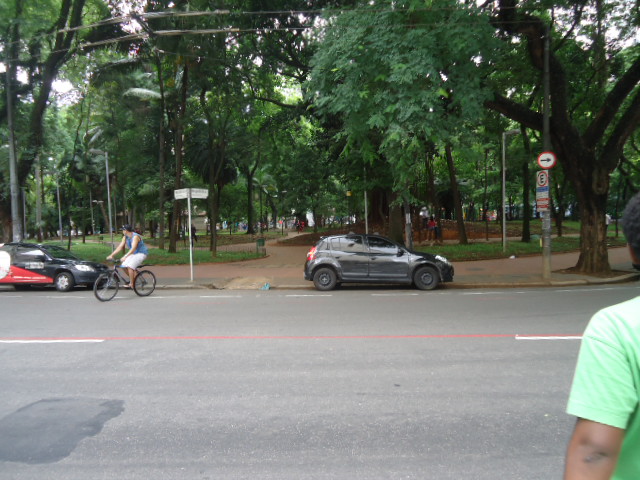This photograph, taken outside on an overcast day, showcases a city park from across a street adorned with a red line down its middle and a couple of dashed white lines. In the bottom right corner, a partially cropped figure in a green shirt is visible. The street features two parallel-parked cars and is lined with power lines. A small dip in the sidewalk leads to a brick path that follows the sidewalk and enters the park. The park itself boasts lush green trees, green islands, several small bushes, and brown sidewalks.